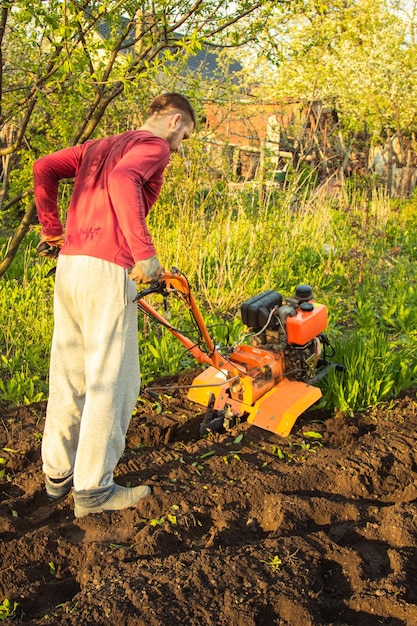This photograph captures a younger man engaged in some gardening work using a rototiller. The man, dressed in a red long-sleeved shirt, grayish-white sweatpants, and sturdy boots, is actively pushing the machine to till the ground. The rototiller is detailed with a red gas tank, a black engine, and orange and yellow fenders protecting the tilling mechanism. The rototiller's handles are a reddish-orange, matching the overall color scheme of the machine. 

The scene is set outdoors on a large plot, previously overgrown with weeds and grasses, now partially tilled as evidenced by the overturned soil where the man has already passed. The remaining ground ahead is still covered in low-growing weeds and grass, indicating the progress he still needs to make. In the background, a rustic building, possibly a barn, stands amidst trees and bushes. Beyond that, a bright, white sky looms over a distant blue mountain range, adding depth to the pastoral setting. The man appears focused on his task, methodically working through the plot to prepare it, perhaps for planting a vegetable garden.